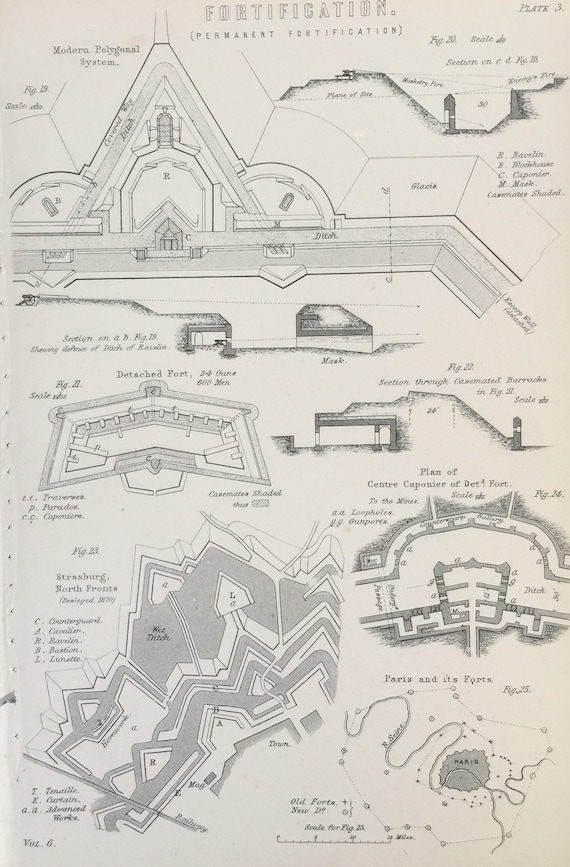This image is a detailed textbook illustration depicting various styles of fortifications. Set against a medium gray background, the black and white line drawings are shaded in gray and arranged in a portrait orientation. At the top of the page, the word "FORTIFICATION" appears in large, uppercase white font with black borders. Beneath this, in smaller uppercase black font within parentheses, is the phrase "PERMANENT FORTIFICATION." To the top right, the image is labeled "Plate 3."

The illustration showcases seven different fortification styles, each presented schematically from a top view, showing intricate details of walls and trench work. Each section is meticulously labeled with minute font, pointing out the different parts. The technical drawings include cross-sections of fortifications from various places and cities, such as Strasbourg in Northern France and Paris. There is also a scale of distance with accompanying text at the bottom right. The overall style is that of a black and white vintage technical illustration, rich in historical and architectural detail.